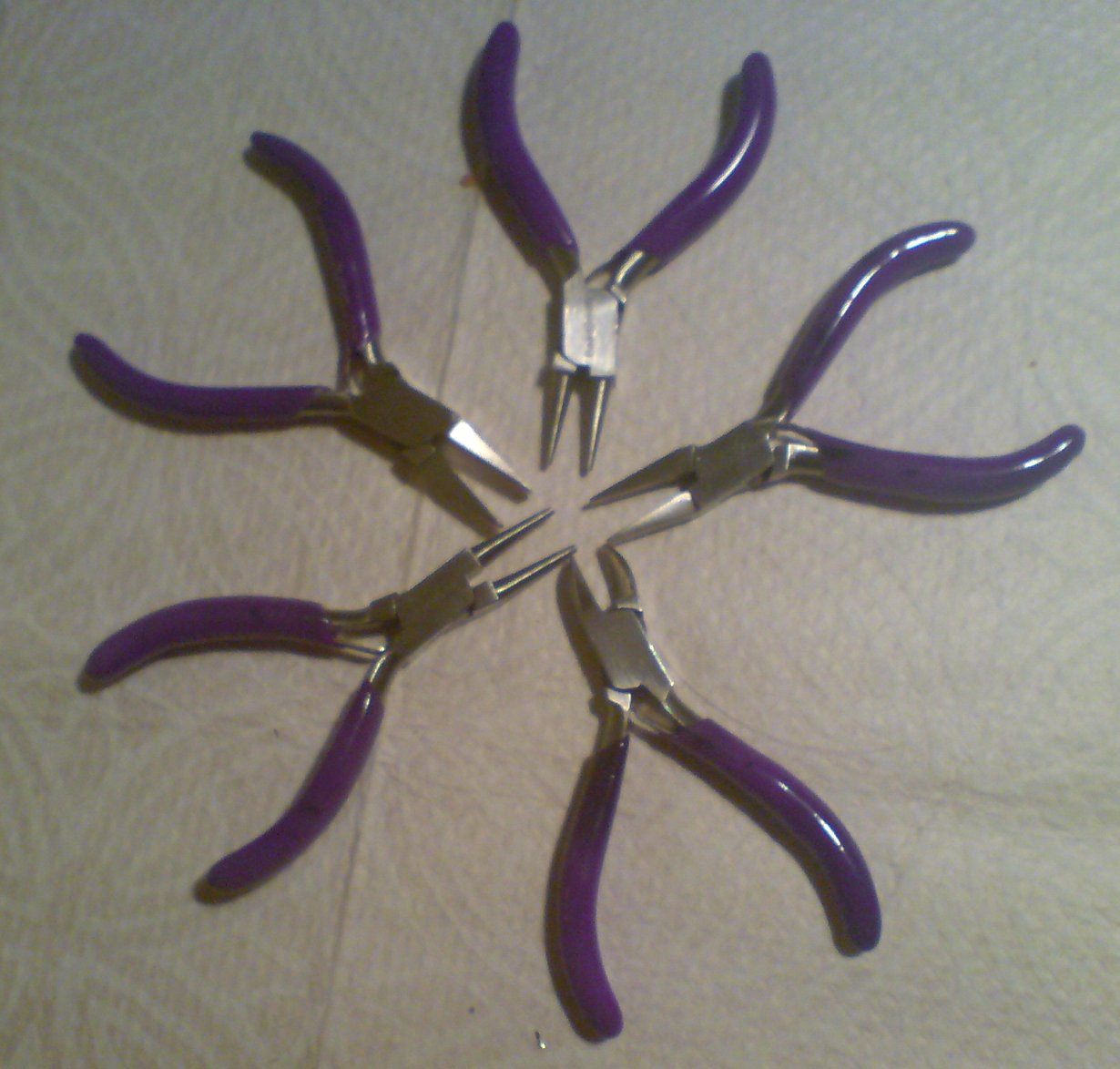In a poorly lit, out-of-focus color photograph, five pairs of pliers with purple, rubbery handles are arranged in a circular formation on a white, quilted-texture paper towel background, creating the appearance of a flower, snowflake, or summoning circle. The silver, steel noses of the pliers point towards the center of the circle, while their slightly open handles fan outwards, resembling petals. Despite the image's low quality, the creative arrangement of the pliers against the contrasting background makes for a visually intriguing composition.